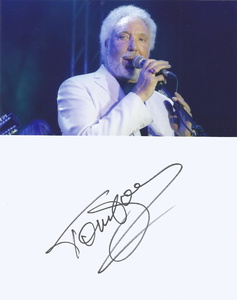The image is a composite of two photographs, with the top half depicting the celebrated singer Tom Jones in the midst of a performance. Tom Jones, who appears to be around 70 years old, is dressed in a long-sleeved white suit jacket and is holding a microphone in his right hand, which also showcases a distinctive ring on his ring finger. He is characterized by his short, white,-gray hair and white beard, and his gaze is directed to the left side of the image, from the viewer's perspective. He has a slight smile and his mouth is open, presumably caught in the act of singing. The background features a blue curtain and a hint of a band member’s instrument on the lower left, though not clearly identifiable.

The bottom half of the image displays a plain white piece of paper with an elaborate, cursive autograph diagonally centered, which reads "Tom Jones," presumably matching the singer in the photo above. This autograph stands out as the only writing visible in this section, maintaining the minimalistic aesthetic that complements the detailed portrait above. The overall composition emphasizes Tom Jones' presence and his signature style.